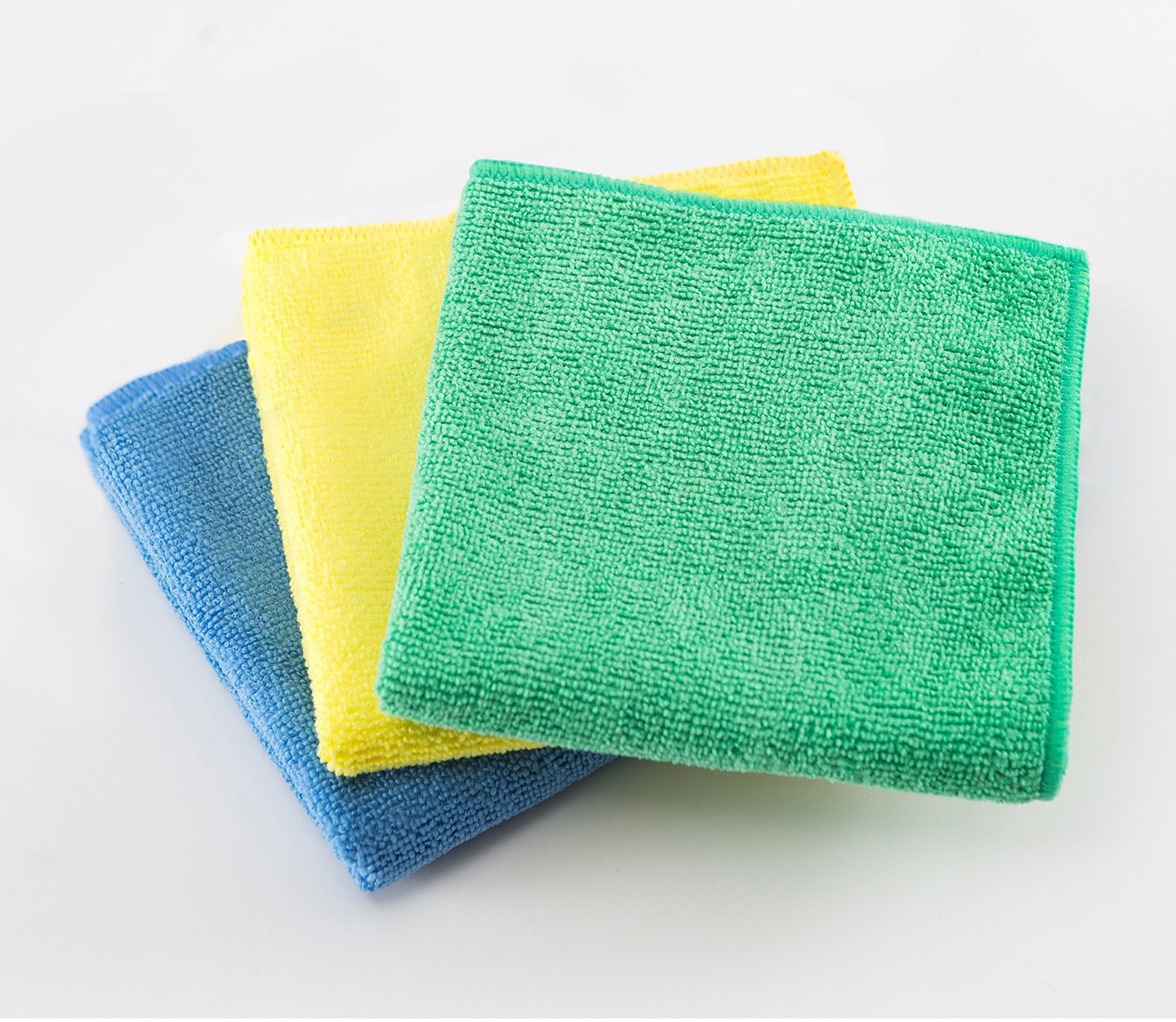This photo showcases three neatly folded microfiber cloths arranged in a fanned-out stack against a very light gray background. From bottom to top, the cloths are blue, yellow, and light green. They are folded into compact squares, allowing the texture of each cloth to be clearly visible. The cloths are clean, either freshly laundered or new, although the green cloth on the top has a slight dark spot on its right side.